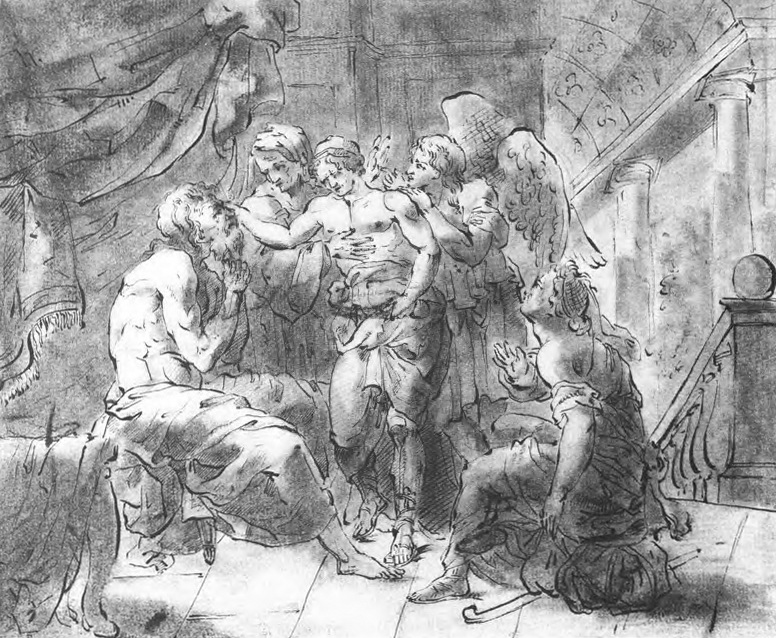This artwork, rendered in a sketchy style using a palette of grays and whites to provide intricate details, features a dramatic central scene. At the heart of the image stands a shirtless man, who is supported on both sides by what appear to be angels, identifiable by the wings of at least the right one. This man, clothed in a toga-like garment and sandals, extends his hand to touch the forehead of a bearded, pleading man seated before him, who has his hands clasped in a gesture of supplication. This seated man has only a blanket or fabric draped over his legs and is barefoot. Beside them is another man, kneeling on the floor with one leg bent, seemingly in a state of worship. To the right, a woman is seated nearby, looking up at the central figure and reaching out, though not directly towards him. They are all situated indoors, as indicated by the discernible railing or staircase, pillars, and drapery in the background, giving the setting a grand, possibly Greek architectural ambiance.